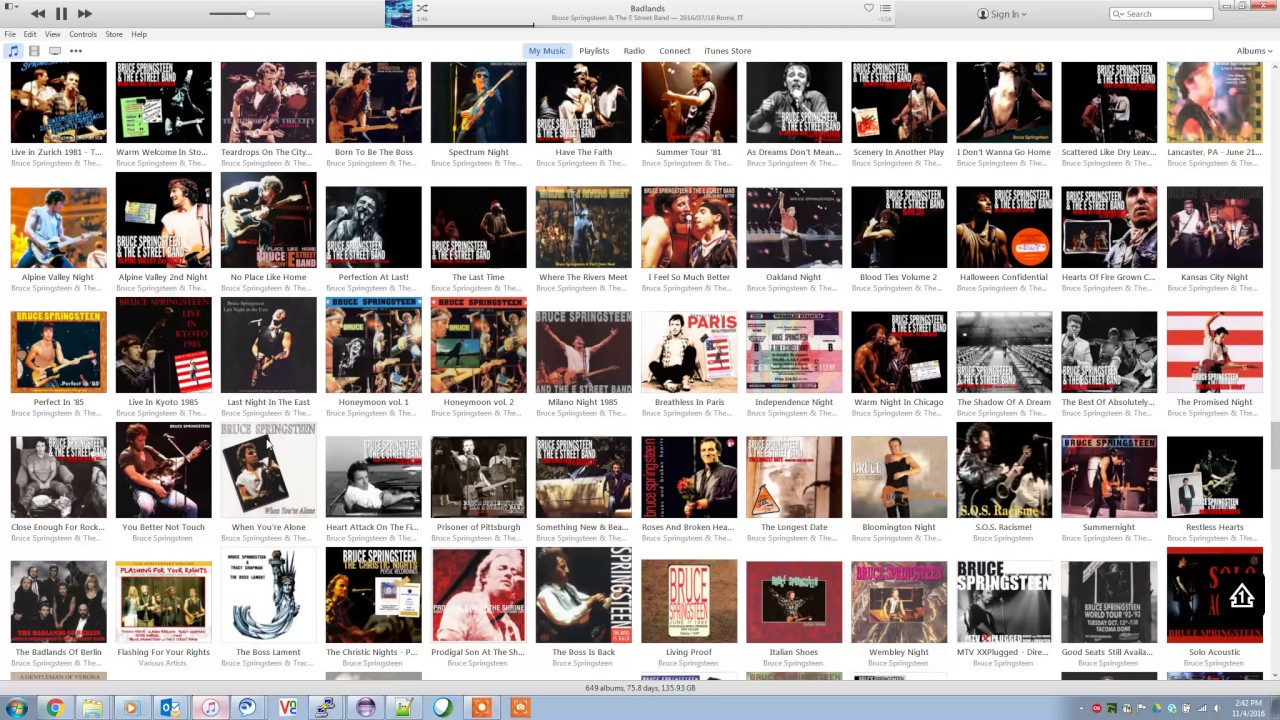A search result displayed on a large 27-inch Apple monitor showcases a grid of 60 image thumbnails, all featuring musician Bruce Springsteen. The monitor screen, likely running macOS, displays various applications, including Apple Music, Google Chrome, and Files. The visible thumbnails include iconic albums such as "Born in the USA" and various live performance covers, offering a comprehensive visual array of Bruce Springsteen's prolific musical career.